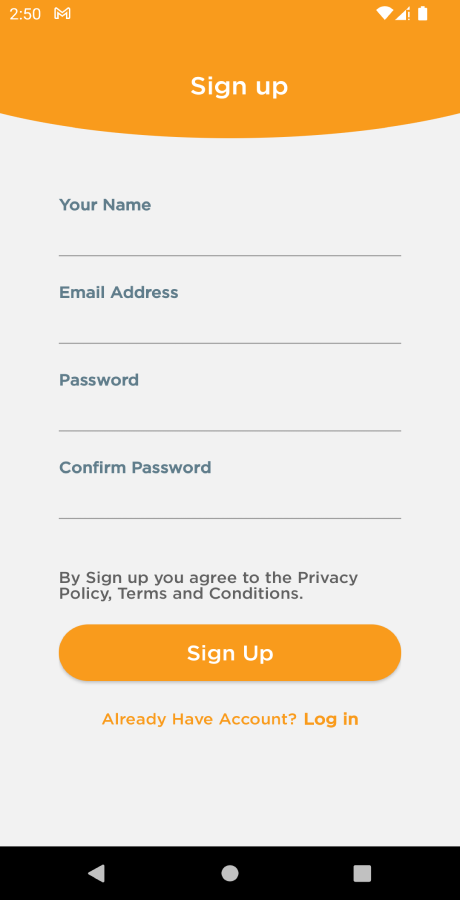The image is a screenshot of a smartphone or tablet interface displaying a sign-up form.

In the status bar at the top left, the time is shown as "14:50," indicating it is set to military time. Next to the time is a Google Gmail icon. On the top right, symbols show a full Wi-Fi signal and an almost full cell phone signal with an exclamation mark next to it, indicating an issue. Also present on the right is a fully charged battery symbol.

The screen features an orange, semi-circular band at the top, within which, on the right edge, bold white text reads "Sign Up." Below this band is a gray, downward-curved rectangle that meets the orange band at the top and is divided into different sections.

The first section in the gray rectangle has a blue header labeled "Your Name," followed by a black line. The subsequent sections are labeled "Email Address," "Password," and "Confirm Password," each followed by a black line, indicating input fields for a sign-up form.

Below the form sections, in black text, it reads, "By signing up you agree to the privacy policy, terms and conditions." This is followed by an orange oval button with white text in the center that says "Sign Up." Lower still, in orange text, it prompts, "Already have an account?" and in bold orange text, "Log In."

At the bottom of the screen is a black bezel containing three icons: a left-turned arrow (gray) for going back, a circle (usually for returning to the home screen), and a square (for viewing and selecting open windows).